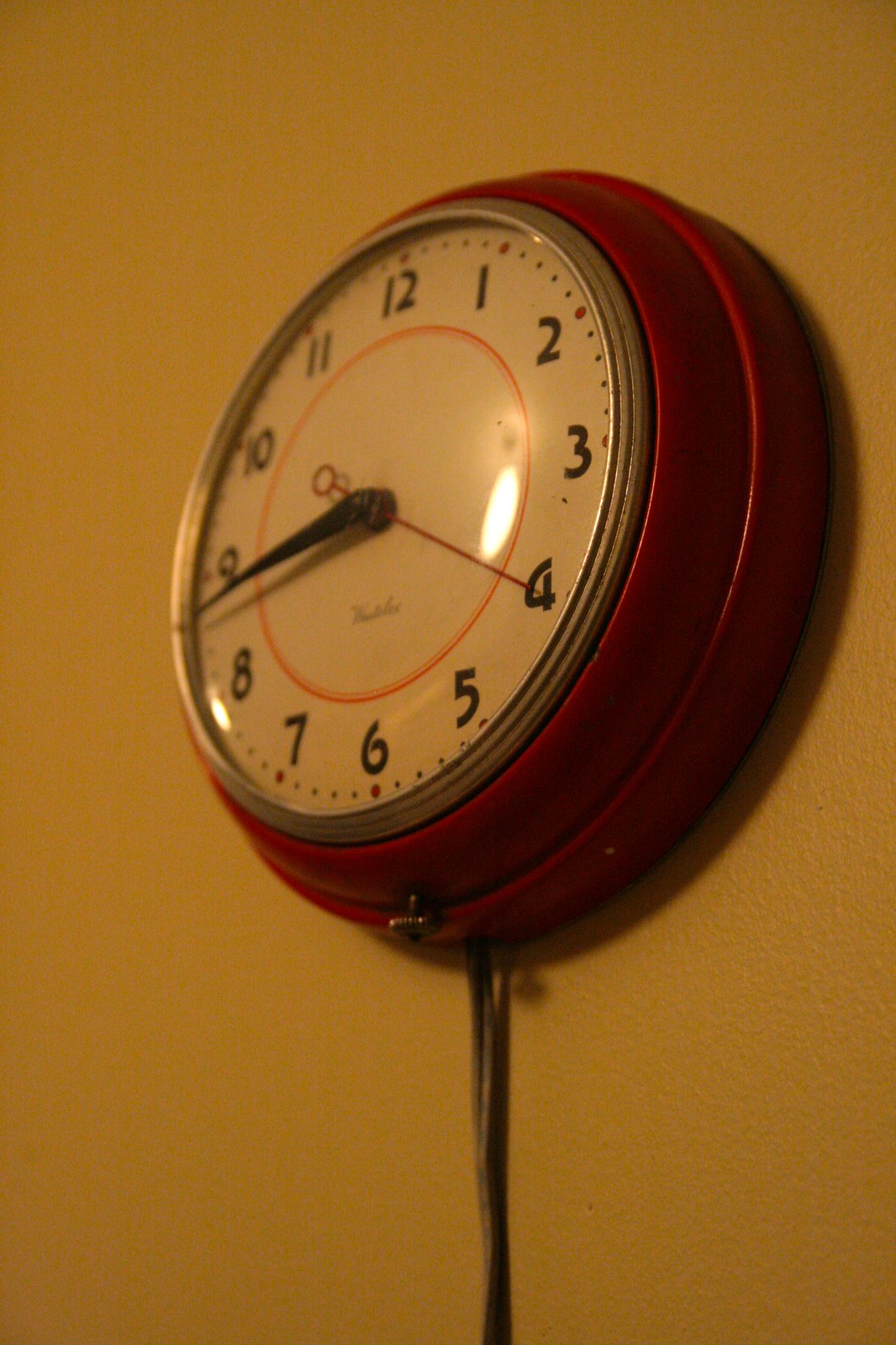A striking photograph, likely taken with a phone, captures an old-fashioned clock prominently displayed on a slightly yellow-painted wall. The vertical orientation of the image emphasizes the clock, which occupies over 70% of the frame and is positioned at the center. This vintage timepiece, reminiscent of those found in training rooms or pools, is angled slightly to the left but primarily faces forward. The clock features a layered design with two protruding red metal sections, making it stand out from the wall. The main face of the clock is an analogue design, encircled by the numbers 1 through 12. At its heart lies an orange ring, accentuating the positions of the clock hands. The larger hand points to the 9, while a slender red hand indicates the 4. A visible cord extends downward from beneath the clock, trailing out of the image's lower boundary.